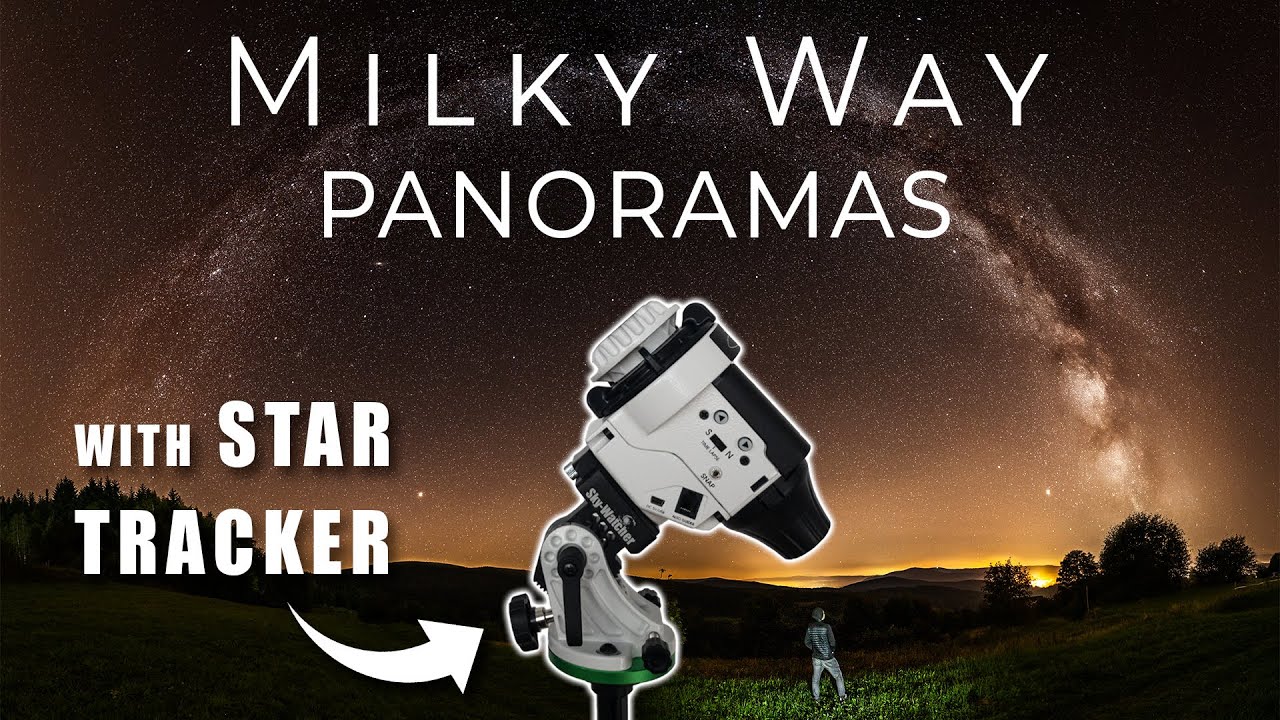The image, resembling an advertisement for advanced astronomical equipment, prominently showcases a sophisticated telescope at its center. This telescope, likely a Cassegrainian type, is characterized by an off-white body with black trim and intricate details such as mounting handles, adjustment knobs, tripod mounts, an SN switch, a sharp adjustment feature, an eyepiece, and a twisted adjustment front lens with finger holds. The background captures a stunning night sky dominated by the Milky Way, vividly illustrating long-exposure stars forming a cloud-like structure, accented by a few prominent stars visible to the naked eye. An amber glow subtly marks the horizon, hinting at the evening's transition to night. At the bottom of the image stands an illuminated man in a black jacket, facing away and gazing upwards, with the text "Milky Way Panoramas" prominently displayed over the starry background. A white arrow points towards the telescope, accompanied by the phrase "With Star Tracker" at the left bottom corner, emphasizing the device's tracking capabilities. The scene is complete with silhouetted trees extending along the horizon, enhancing the depiction of this captivating night sky observation.